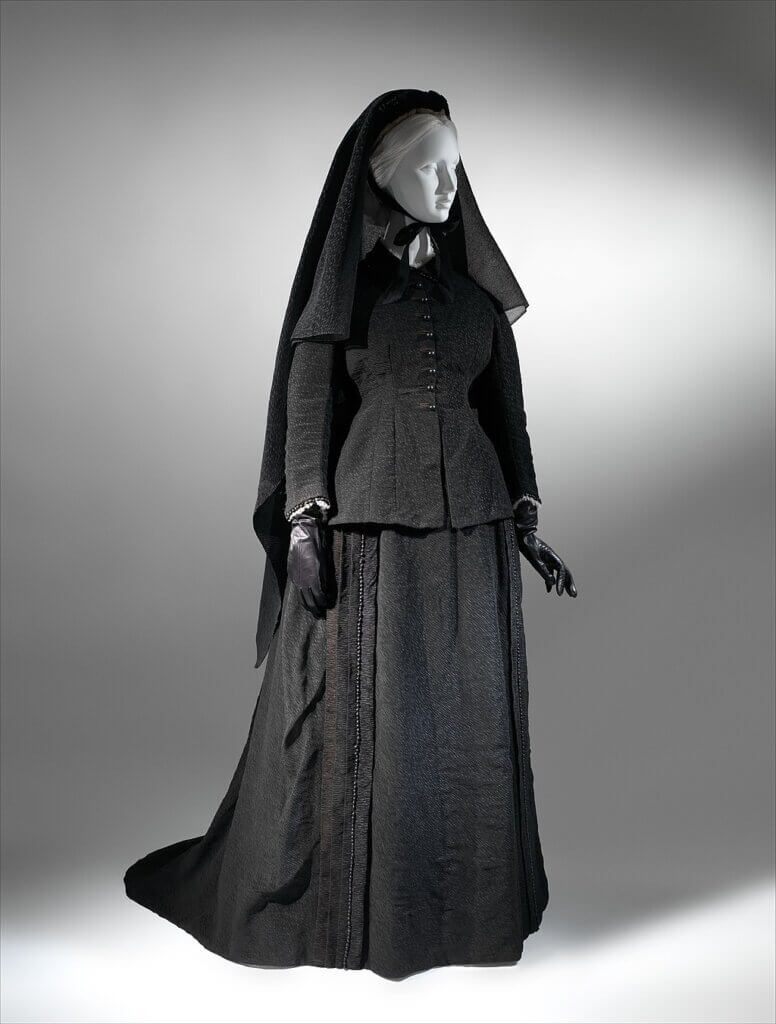This black and white image features a mannequin of a woman dressed in an elaborate vintage mourning outfit, reminiscent of mid-1800s fashion. The mannequin has a pale white face and similarly colored hair, starkly contrasting with her entirely black attire. She is adorned with a long, flowing black veil that drapes from a bonnet and extends well past her waist, almost down to her knees. The outfit includes a long-sleeved, button-up black top that conceals all but a glimpse of a white shirt beneath it. Her hands are covered in dark black leather gloves, and she wears a voluminous black skirt that reaches the floor and trails behind her. The mannequin is positioned in front of a white and gray background, with dramatic lighting casting dark shadows across the rear wall, enhancing the somber and vintage feel of the scene.